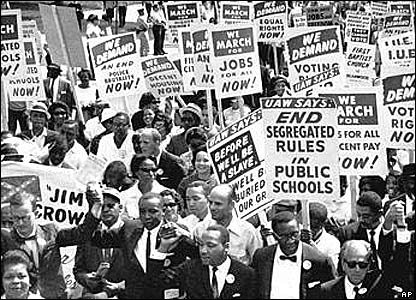The black-and-white image depicts a protest scene from the 1960s, centered around Martin Luther King Jr., who is seen at the bottom center of the image with his hand raised, possibly giving a speech. The predominantly African American crowd, including a few white individuals, marches shoulder-to-shoulder, many dressed in suits and ties, holding rectangular signs that convey powerful messages. Some of the legible signs read "UAW says end segregation rules in public schools," "We demand an end to police brutality now," and "Jobs for all now." The atmosphere is tense, indicated by the distant presence of policemen standing to the side, observing the marchers. This protest, likely during the Jim Crow period, visually captures the fervor and demands for civil rights and equality.